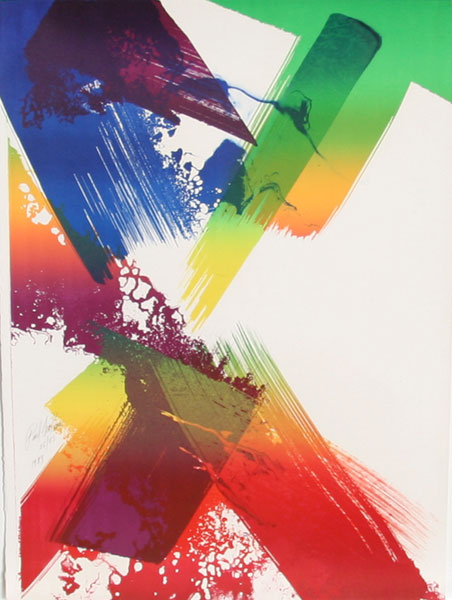This abstract painting, depicted in a photo, features a dynamic symphony of colors against a white background. Dominating the scene are bold geometric shapes and thick brush strokes that intermingle to create a vibrant composition. In the top left corner, a blue rectangle with fringes extends diagonally towards the image's midpoint, overlaid with splashes of purple. Adjacent to the blue form, an orange triangle points in a similar direction. To the right, a green and orange cross ascends from the bottom left to the top right, its center interspersed with a smaller, multi-hued rectangle in shades of dark green, light green, and yellow. The center is marked by a broken purple rectangle with squiggles at its ends. Another diagonal shape, in orange and red with green fringes, rises from the bottom right aiming towards the top left. Red swatches are present at the bottom, sometimes mingling with purple, yellow, and green. The middle left and bottom right sections showcase cloud-like formations, adding texture to the scene. A solid green stripe ends mid-page, accompanied by another thick brush stroke. Splotches of orange, yellow, and purple appear sporadically around these main elements, enhancing the intricate interplay of colors and forms within this contemporary, modern artwork.